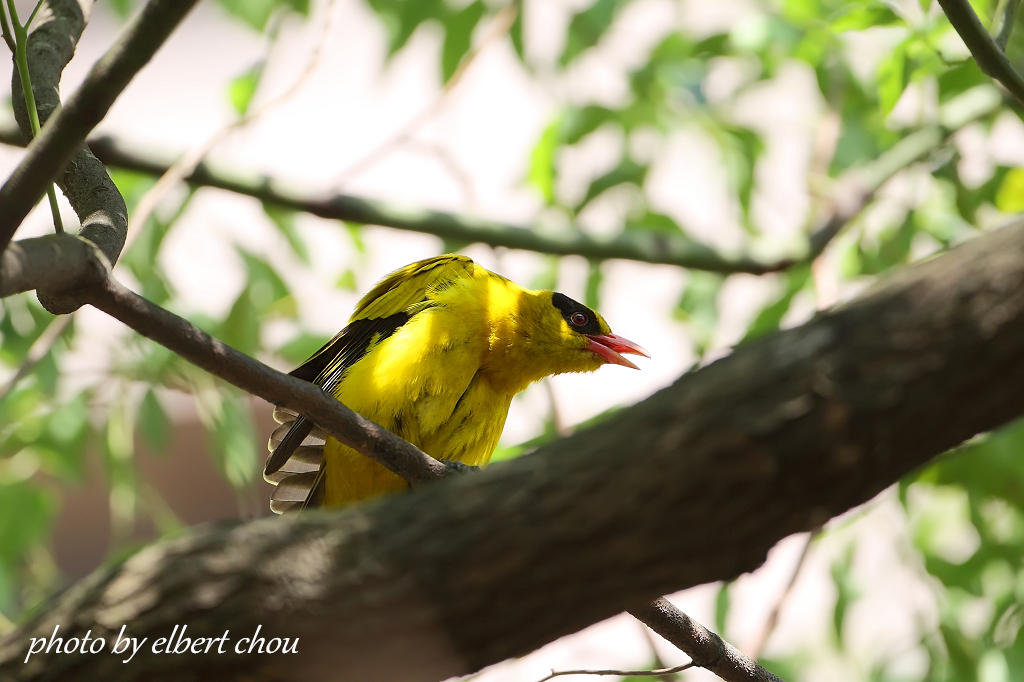This image captures a vibrant scene outdoors, likely taken in the middle of the day, featuring a striking black-naped oriole perched on a robust tree branch positioned diagonally from the bottom left to the center of the frame. The bird, predominantly yellow with a distinctive black stripe on its head and black feathers on its back, is shown with its beak open, possibly chirping. This close-up shot allows us to see the rough texture of the grayish branch and hints at another branch extending sideways in the distance.

The background of the image is blurred, creating a bokeh effect that emphasizes the bird and the branch while suggesting a natural setting filled with leaves and possibly other trees. The colors in the photograph include green, brown, yellow, orange, black, and tan, enhancing the naturalistic feel of the scene. There is a piece of fencing resting on the branch, adding an unexpected element to the composition.

Text at the bottom left corner of the image reads "Photo by Albert Chu," confirming the photographer. This photograph, rich in detail and color, appears to be a snapshot taken by an avid birdwatcher, capturing a serene moment in nature.